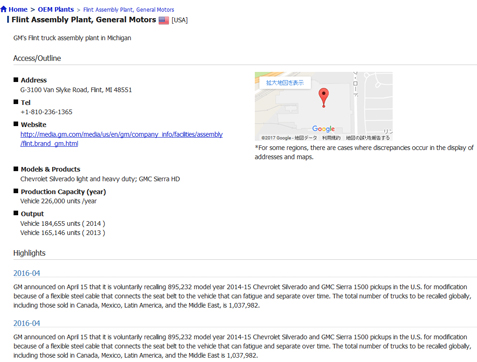**Detailed Caption:**

This image is a screenshot from a document detailing various attributes of the Flint Assembly Plant operated by General Motors in Flint, Michigan. The document's header reads, "Home OEM Plants, Flint Assembly Plant General Motors," indicating that this is an informational page about the facility. On the right side of the document, a Google Maps shot displays the location of the Flint Assembly Plant. Interestingly, there are some Asian characters adjacent to the map image.

The document provides specific details about the plant, such as the address, telephone numbers, and the website link for further information. Additionally, it lists the models and products manufactured at this location, specifically the Chevy Silverado light and heavy-duty trucks.

Production data for the facility is specified, highlighting a production capacity of 226,000 units per year, with an actual output of 184,000 vehicles in 2014. Historical data points to a production output of 65,000 vehicles in a previous year, 2013.

At the bottom of the document, there's a section labeled "Highlights," which includes notable incidents such as a voluntary recall announced by GM in April 2016. The recalls detailed cover unspecified models, indicative of standard public information dissemination about the plant's operations and historical performance.